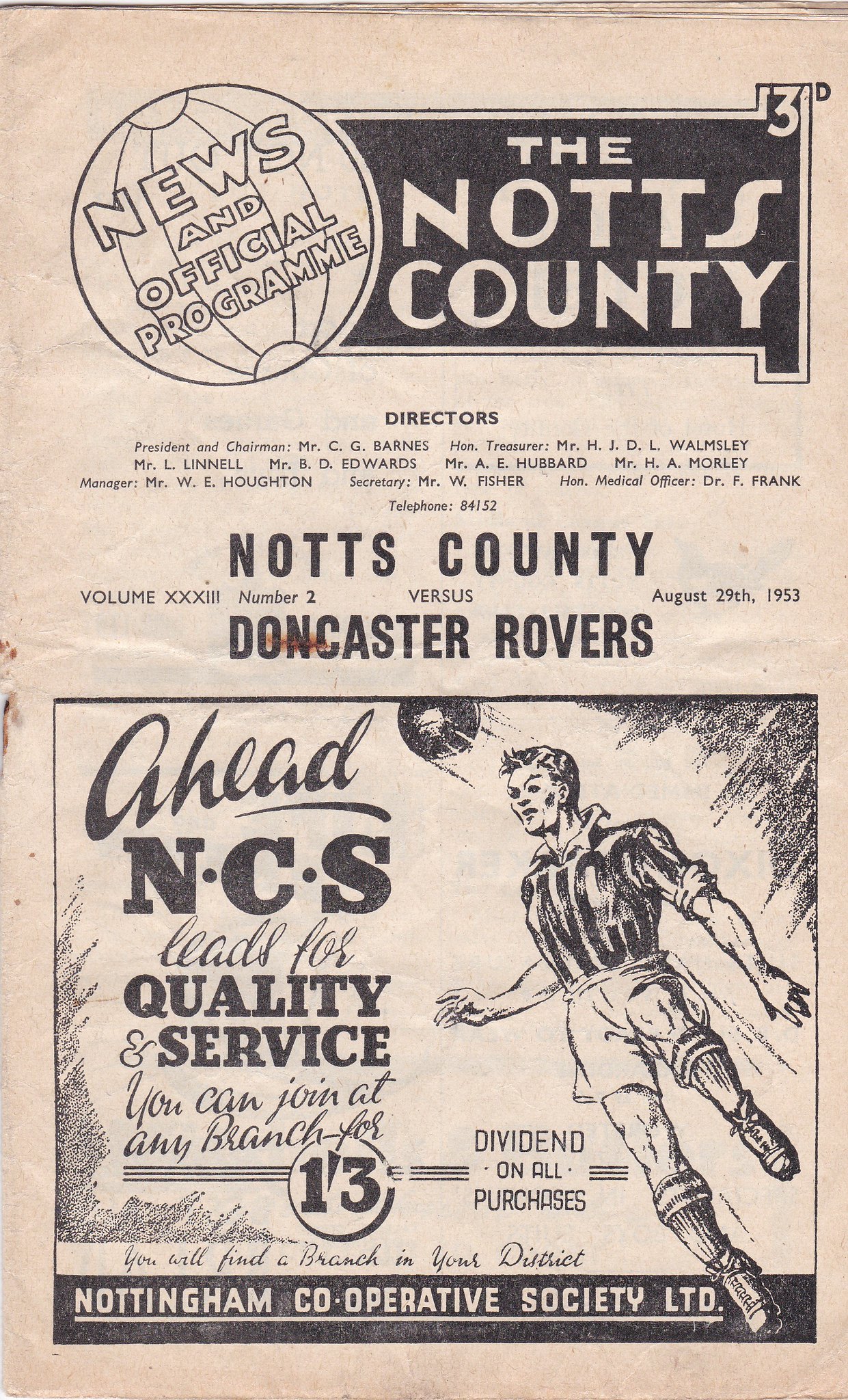The image is a detailed vintage print cover from a soccer club program, dated August 29, 1953, for a match between Knott's County and Doncaster Rovers. The page is printed in black on a light brown background, with prominent black and white elements. At the top left, there's an outline of a globe with the angled text "News and Official Program" superimposed over a horizontal black rectangle. Below, larger white text reads "Knott's County," followed by "Directors" and a list of names and titles including President and Chairman Mr. C.G. Barnes, Home Treasurer Mr. H.J.D.L. Wadsmele, Mr. L. Linen, and Mr. P.M. Edwards. The lower half of the page features an advertisement for the Nottingham Cooperative Society Limited, highlighted by a line-art illustration of a soccer player heading the ball, with the text "Ahead NCS Leads for Quality Service. You can join any branch." The player's shirt has "NCS" written on it, reinforcing the sponsor's message. The overall style evokes a nostalgic feel typical of mid-20th-century sports publications.